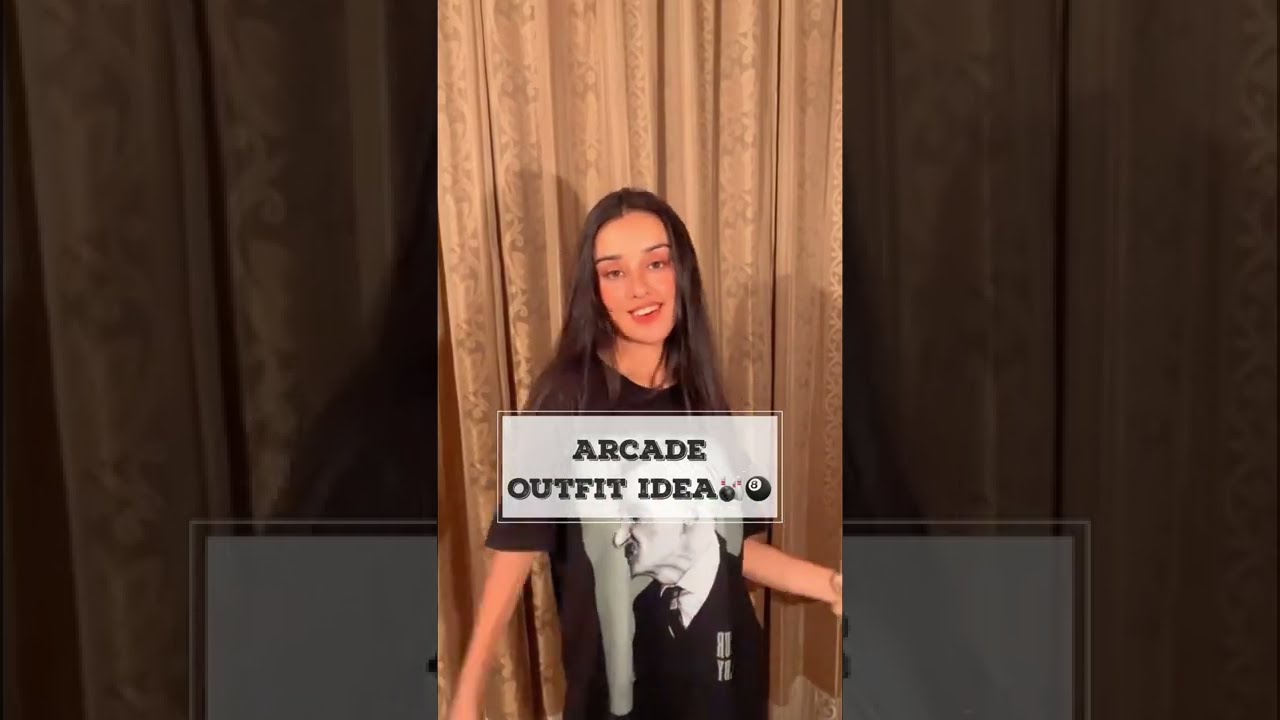The image is a vertically-oriented cell phone photograph, with an enlarged and darkened version of the same image used as a faded background on both the left and right sides, creating a unique framing effect. In the foreground, a young Caucasian woman stands in front of long, gold or brown-colored curtains. She has straight, dark brown hair parted precisely down the center, which cascades past her shoulders. Facing the camera with her head slightly tilted to the side, she displays a half-smile, showing her upper teeth, and her thin brown eyebrows frame her expression. 

Her attire comprises a very large black T-shirt, which could also be mistaken for a shirt dress due to its oversized fit. The shirt features a black-and-white image of an older white man, possibly a military general or politician, dressed in a suit. A gray rectangular box, laid out in landscape orientation and centered on her chest, contains two lines of bold black text reading "Arcade Outfit Idea," accompanied by a small magic 8-ball symbol. The woman’s arms are extended to the sides, and her body is slightly turned at the hips, suggesting she might be dancing. The combination of her dynamic pose and the creative use of the background enhances the central image, making it stand out prominently.